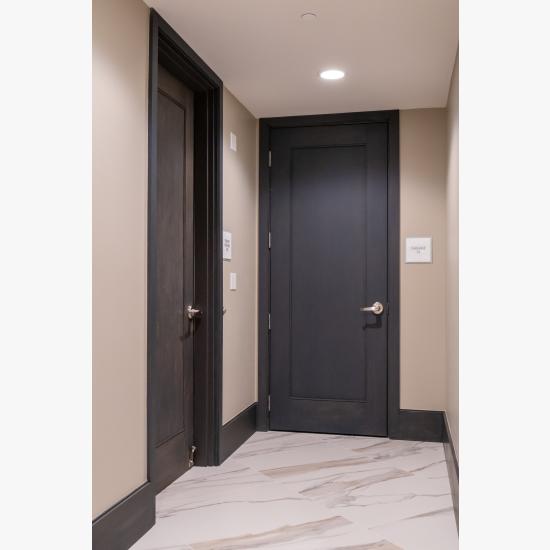This detailed photograph captures the end of a hallway in either an apartment or a hotel building. The hallway features a pristine, polished stone tile floor, with the tiles predominantly white and tan in color, interspersed with subtle brown patches and designs. The corridor is bordered by light tan walls and a white ceiling, enhancing the space's bright and neutral aesthetic.

At the far end of the hallway, there are two wooden doors: one on the left and one on the right wall. The door on the left is a dark brown hue, while the door on the right is an even deeper brown, almost black. Both doors are single-panel hardwood with shiny metal handles positioned towards the bottom part of each door. The doors are flanked by white square plaques, possibly indicating room numbers or names, although the text is too small to discern.

In the upper center of the hallway ceiling, a white circular light fixture casts a bright, even illumination throughout the space. Also visible on the walls near each door are white light switches, adding functional detail to this well-lit and meticulously maintained hallway, designed to provide clear and inviting access to the rooms at the end.